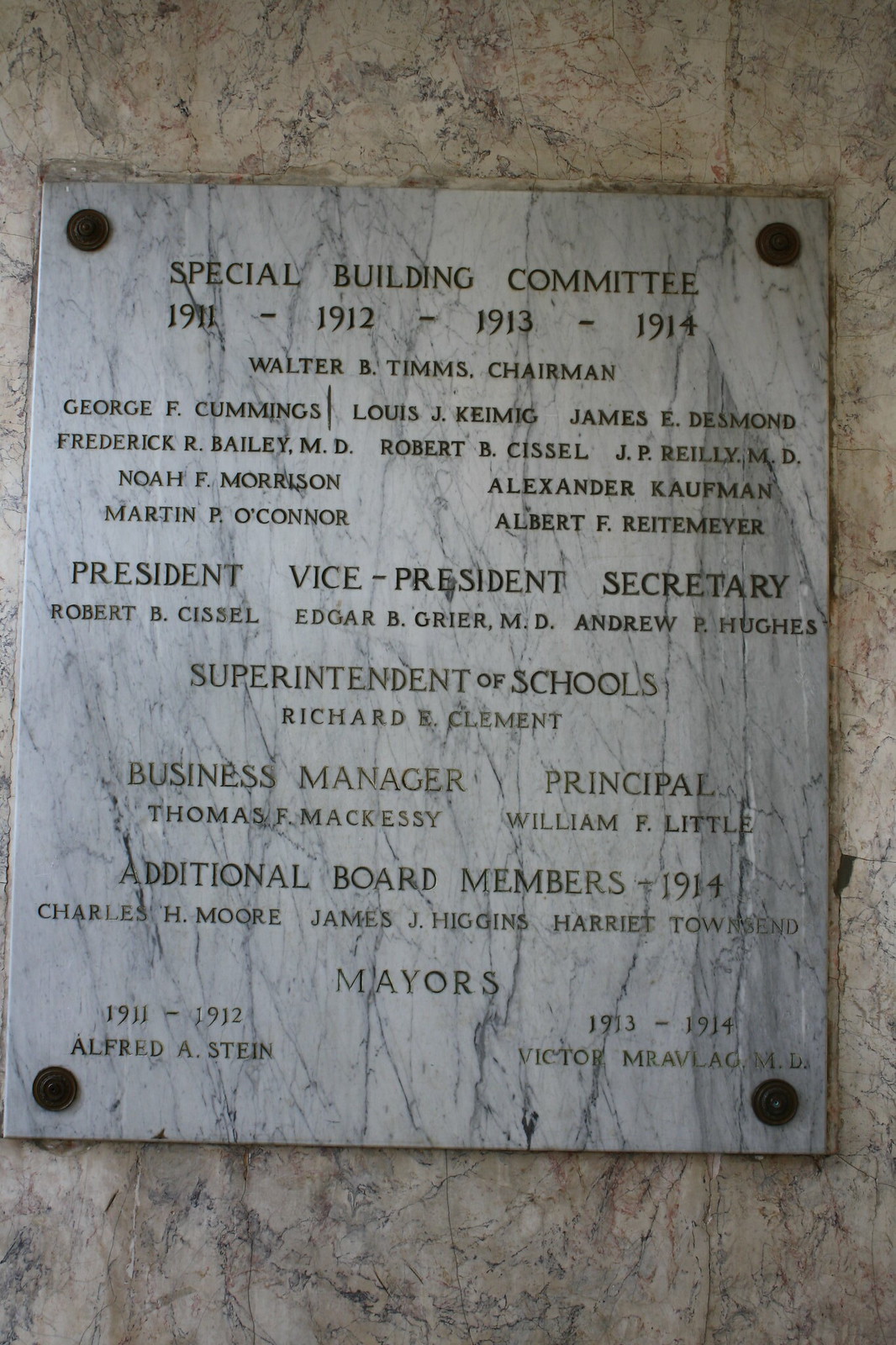This image showcases a detailed building plaque mounted on a polished white marble background with intricate black marbling and cobweb-like patterns. The plaque, affixed with rivets in all four corners, is slightly whiter than the marble it is attached to. At the top, it prominently reads "Special Building Committee" in bold black letters, followed by the years 1911, 1912, 1913, and 1914, indicating the period during which the committee was active.

The committee chairman, Walter B. Timms, is listed prominently beneath the date range. The plaque meticulously catalogs the names of various committee members, including George F. Cummings, Louis J. Kamig, James E. Desmond, Frederick R. Bailey, Robert B. Sissel, J.P. Reilly, Nora F. Morrison, Alexander Kaufman, Martin P. O'Connor, and Albert F. Reitmeyer. Each name represents a significant contributor to the committee.

Additionally, the plaque identifies key positions such as president Robert B. Sissel, vice president Edgar B. Greer, M.D., and secretary Andrew B. Hughes. Furthermore, it lists the superintendent of schools, Richard D. Clement; business manager, Thomas F. McKissie; and principal, William F. Little, highlighting their roles in maintaining and managing the educational and administrative functions during those years.

Finally, it acknowledges the mayors serving during the committee's tenure: Alfred A. Stein (1911-1912) and Victor Relavig, M.D. (1913-1914). This plaque serves as a historical record of the individuals who played a pivotal role in the building committee's activities and the governance of the community during those formative years.